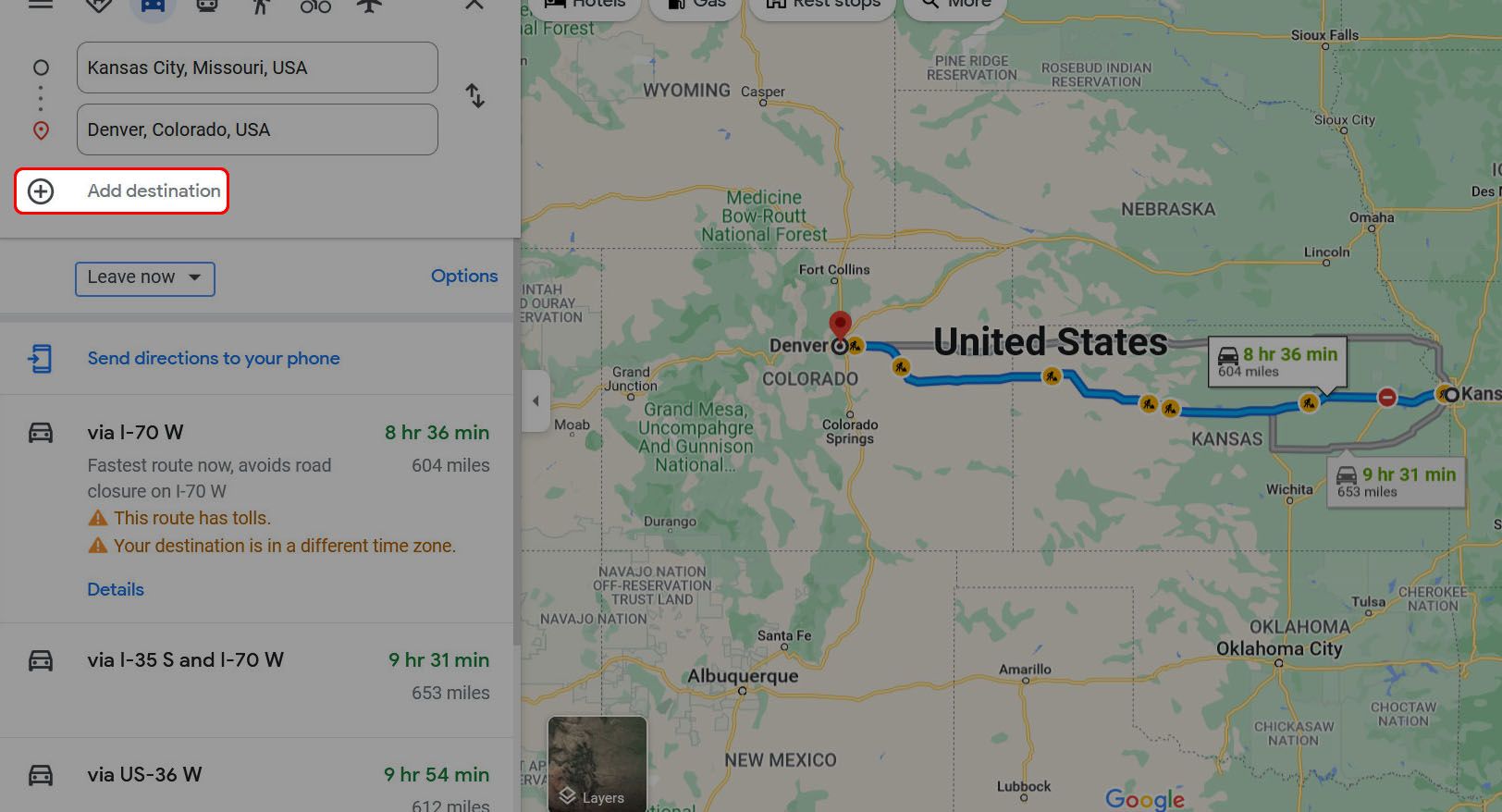The image displays a Google Maps screen with a route mapped out from Kansas City, Missouri, to Denver, Colorado. The primary route, highlighted in blue, follows I-70 West, covering a distance of 604 miles and estimated to take 8 hours and 36 minutes. Alternative routes are also visible: one via I-35 South and I-70 West, encompassing 653 miles and taking approximately 9 hours and 31 minutes, and another via I-36 West, spanning 612 miles with an approximate driving time of 9 hours and 54 minutes. 

On the left panel, options are available to add destinations and send directions to a phone. The overall map of the United States forms the background, with the specified route prominently outlined. A key feature in this image is a red box around the "Add Destination" button, which is grayed out and dimmed, emphasizing the tutorial aspect of adding stops to an itinerary. This instructional element highlights the ease and usefulness of incorporating multiple destinations into trip planning on Google Maps.